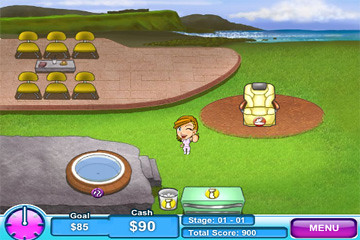This image appears to be a screenshot from an animated game. At the bottom of the screen, there is a blue bar displaying a clock or timer, accented with purple. Accompanying this timer is a goal indicator, stating a target of $85, with the current cash showing $90, indicating the goal has been surpassed. Adjacent to the timer, it reads "stage-01-01" with a "total score" of 900 displayed beneath it. Further right, there is a purple button labeled "menu."

The main portion of the image showcases a vibrant green field, centrally featuring a cartoon character with a disproportionately large head compared to her body, emphasizing its animated style. In the lower-left corner of the screen, a rock can be seen with a blue, wooden-like pole standing next to it.